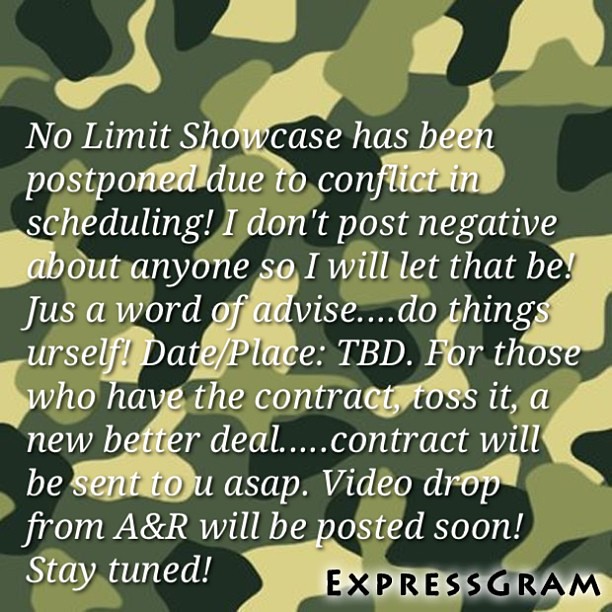This graphic features a camouflage background in shades of dark green, light green, and tan. Overlaid on the camo pattern is a message written in white text, detailing information about a postponed showcase. Key details include a note about the change in scheduling to be determined (TBD) for contract holders, and a reminder for individuals to pursue better deals, with contracts to be sent ASAP. Additionally, there is an announcement about an upcoming video drop from A&R, advising viewers to stay tuned. The text also contains a piece of advice incorrectly spelled as 'advise.' At the bottom right, "EXPRESSGRAM" is prominently displayed in all capital letters with a white shadowy effect, adding a distinct branding element to the graphic.